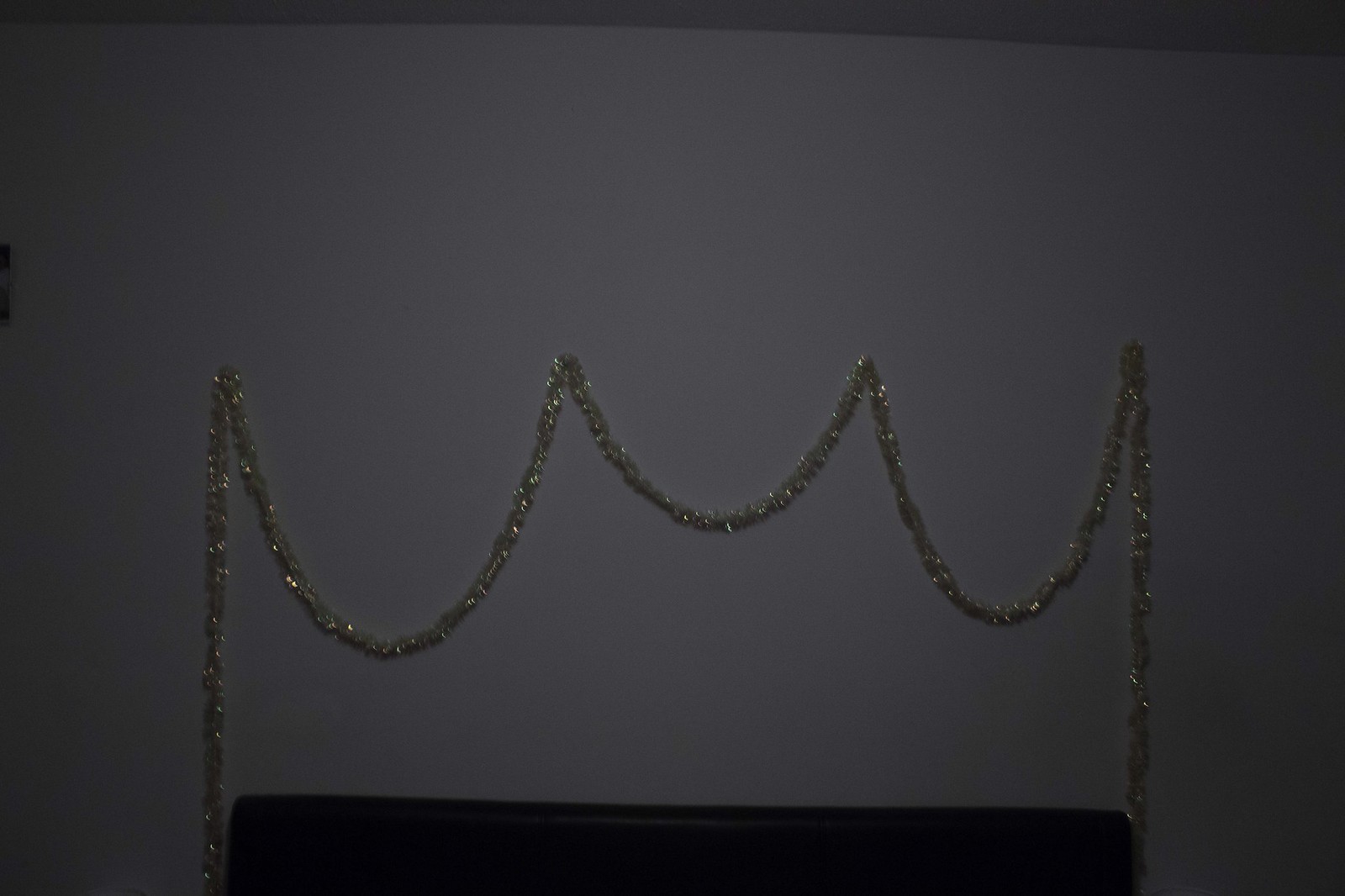The photograph captures a dimly lit indoor scene featuring a white wall backdrop, which appears darker due to the lighting. On the bottom of the image, there is a brown counter or platform, possibly the top of a couch. Hanging on the wall is an elaborate decoration made of gold, sparkly garland, reminiscent of tinsel typically used for Christmas trees. This garland is arranged to create a crown-like shape with two vertical strands on either side. The garland starts from metal rods or pins on each end, rising and forming a large U-shape dip in the center before being pinned back up higher to create a smaller U-shape, then descending again to be pinned in a final U-dip on the right side. The repetitive looping and pinning create a visually striking crown pattern on the wall, adding a festive touch to the setup.